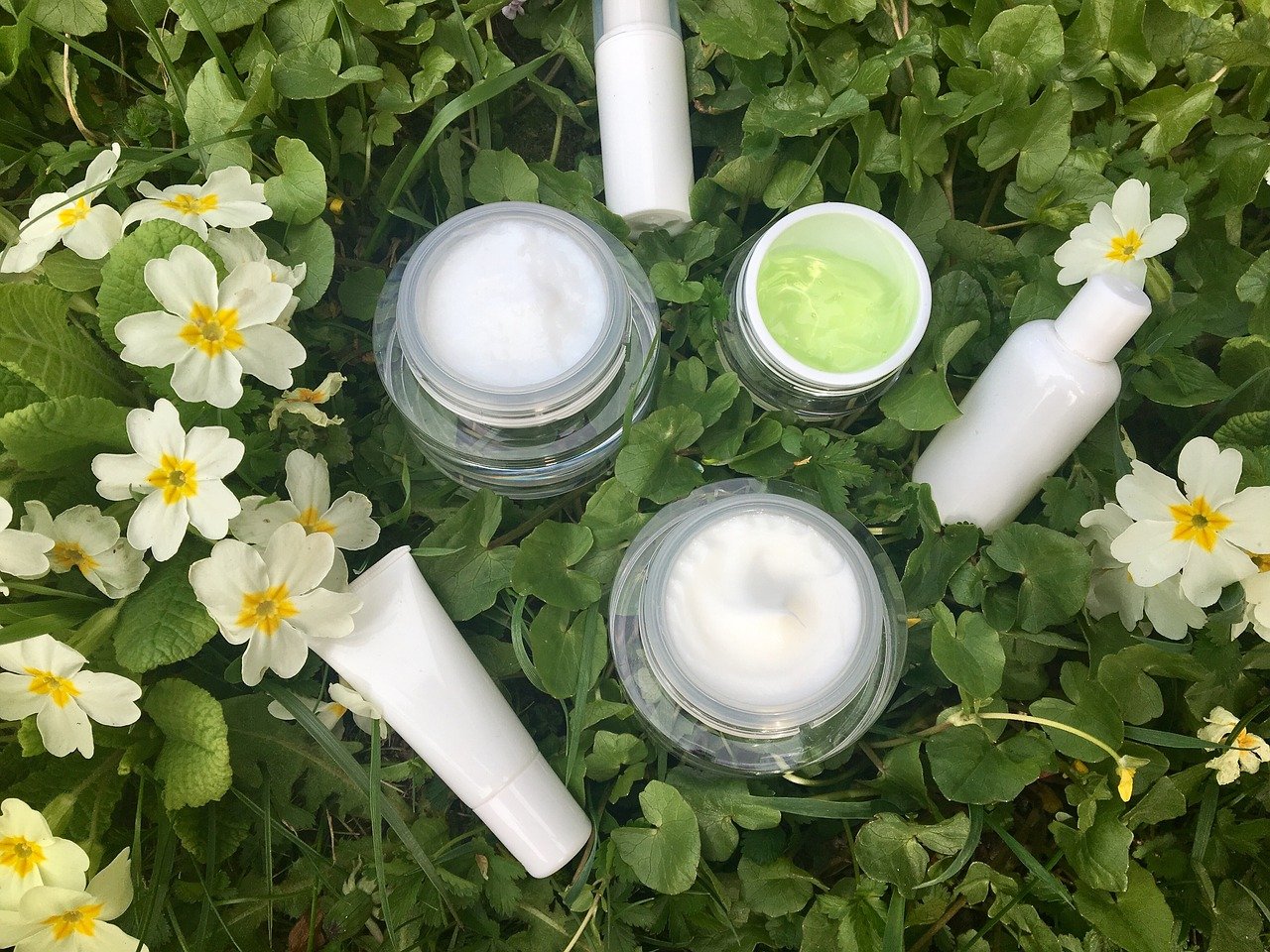This meticulously staged photograph showcases an array of skincare products set against a lush backdrop of green leaves and plants, which appear to be real. Dominating the left side of the frame are clusters of white flowers with vibrant yellow centers, contrasted by a few scattered blooms on the right. The composition features three white, logo-free bottles and three transparent jars, tastefully arranged among the foliage. 

In the bottom-left corner, a squeeze bottle is prominently visible, while the upper-right corner houses a capped bottle. Slightly off-frame, a spray bottle peeks into view. Among the jars, two are larger and contain a rich white cream, whereas the third, slightly smaller jar holds a light lime-green cream. 

The absence of branding gives the scene a minimalist, natural allure, as though someone carefully curated these elements within a green utopia, awaiting the final touches of logos during post-production.